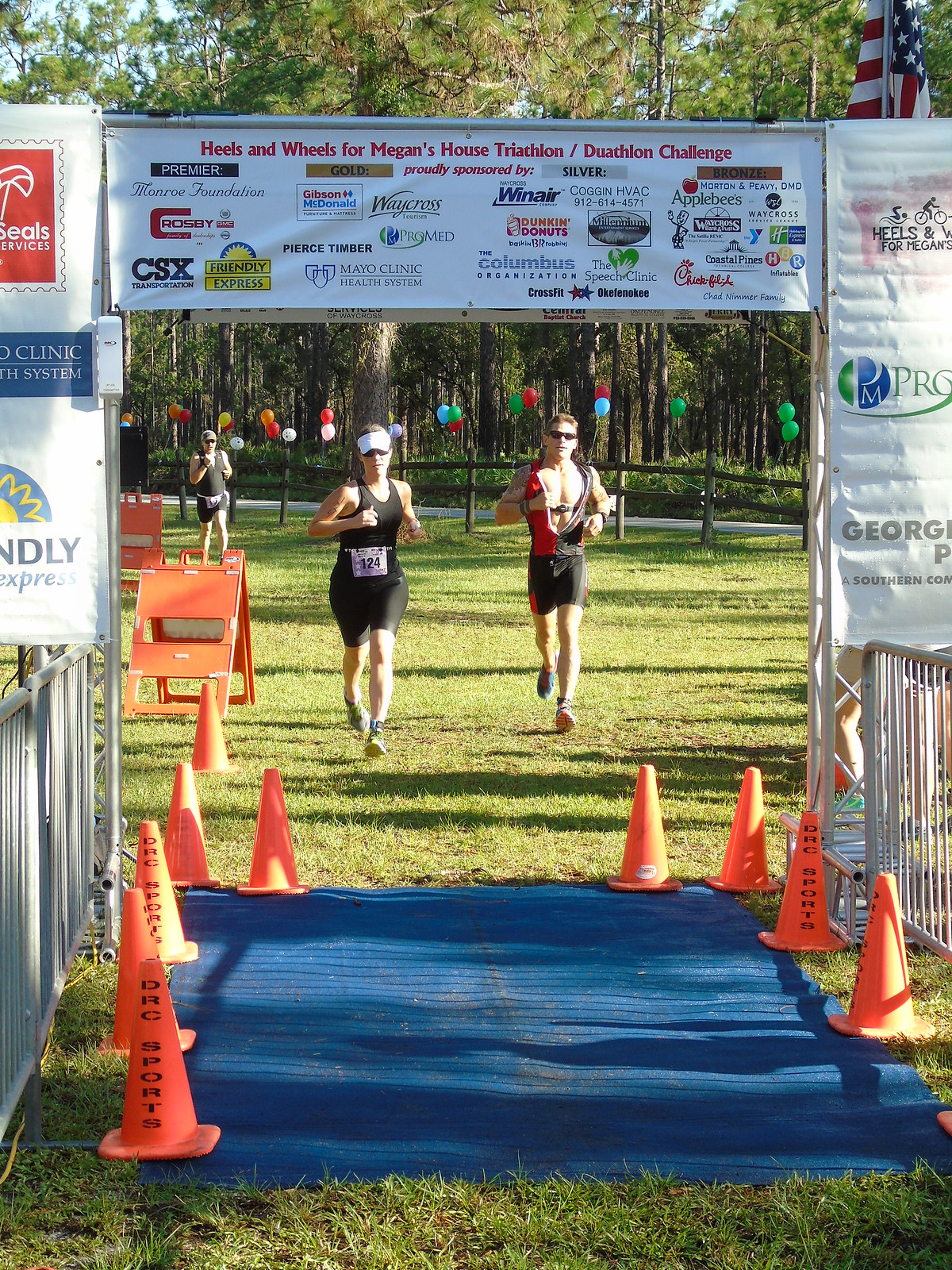The image captures the climactic moment of the "Heels and Wheels for Megan's House Triathlon/Duathlon Challenge," taking place on a grassy terrain. At the center of the photograph, two runners—a woman in a black blouse, black shorts, and a white visor, and a man wearing a red t-shirt and black pants—are approaching the finish line. There's a third runner, a woman approximately 30 feet behind them, also visible in the frame. The finish line itself is marked by a long blue rectangular mat, flanked by orange cones and silver railings that form an entryway. Overhead, an archway bearing the event’s name also showcases advertisements from various sponsors, including Mayo Clinic, CSX Corporation, Dunkin' Donuts, and Chick-fil-A. An American flag can be seen hanging from the top of the right post of the archway. The scene is lit by morning sunlight, which filters through the trees and highlights a wooden fence that separates the forested background from the race area. The atmosphere suggests a well-organized charity event, bringing together participants and supporters for a meaningful cause.